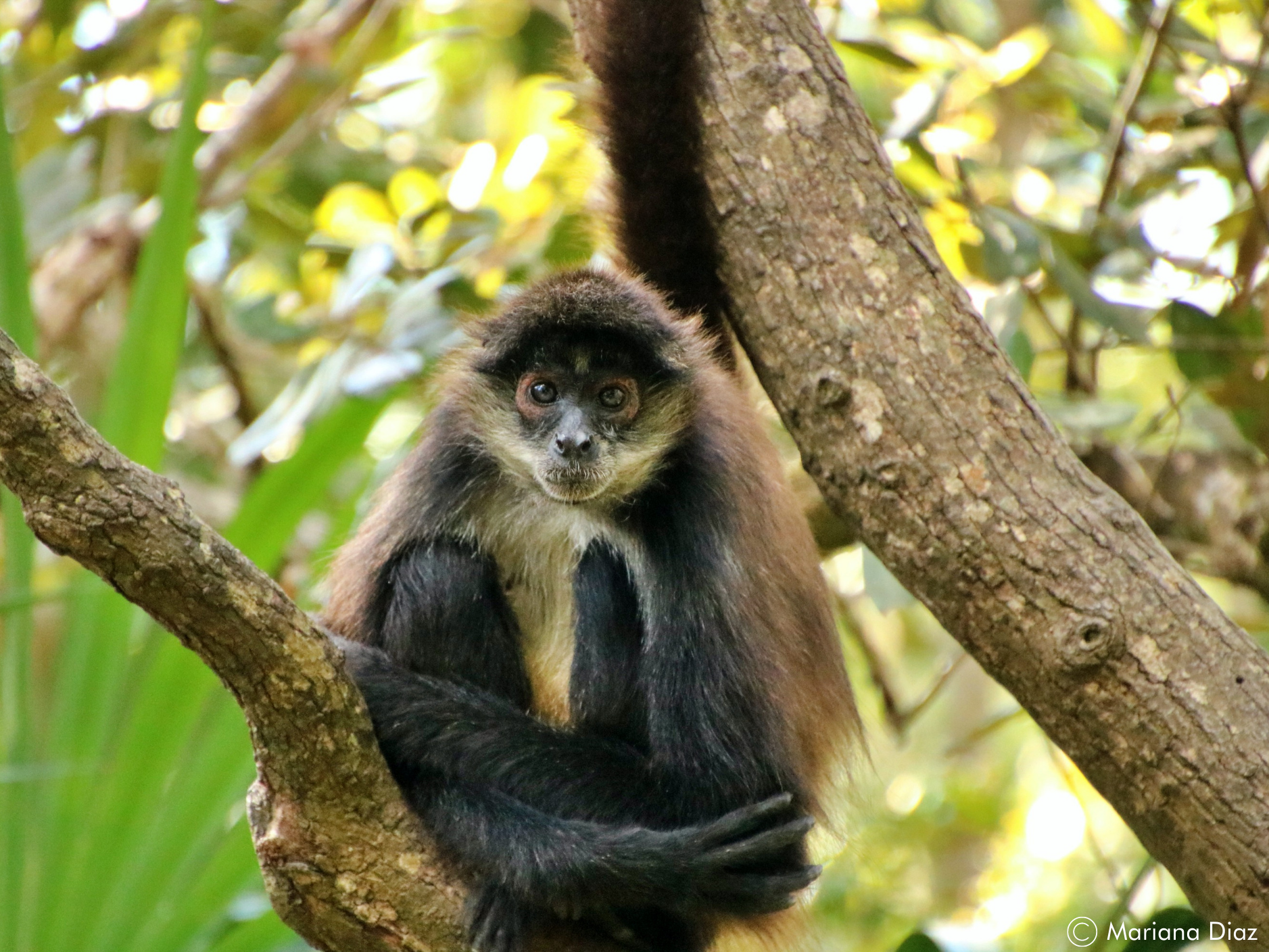The photograph captures a visually striking monkey perched on a tree branch, positioned in the center of a vertically framed, nature-rich image. The focused, close-up view reveals intricate details of the monkey, showcasing its unique appearance. It flaunts long, brown-blonde hair with distinguishing black eyebrows and eyes, encircled by orange rings. Its facial features include a small nose and exposed teeth framed by white fur extending to its chin and neck. The rest of its body is predominantly cloaked in black fur, with black legs and arms. The monkey's posture is relaxed, sitting with its knees drawn close to its chest and arms wrapped around them, almost forming a peace sign with its fingers. It's set against a backdrop of blurred foliage and flowers, interspersed with dappled sunlight filtering through the greenery. Two prominent brown branches support the monkey, one rising from the bottom right corner and another from the bottom center, stretching diagonally across the frame. The background features a mixture of light and dark green leaves, with hints of blue sky peeking through. The image is subtly marked with the copyright text "Marina Diaz" in white at the bottom right corner.